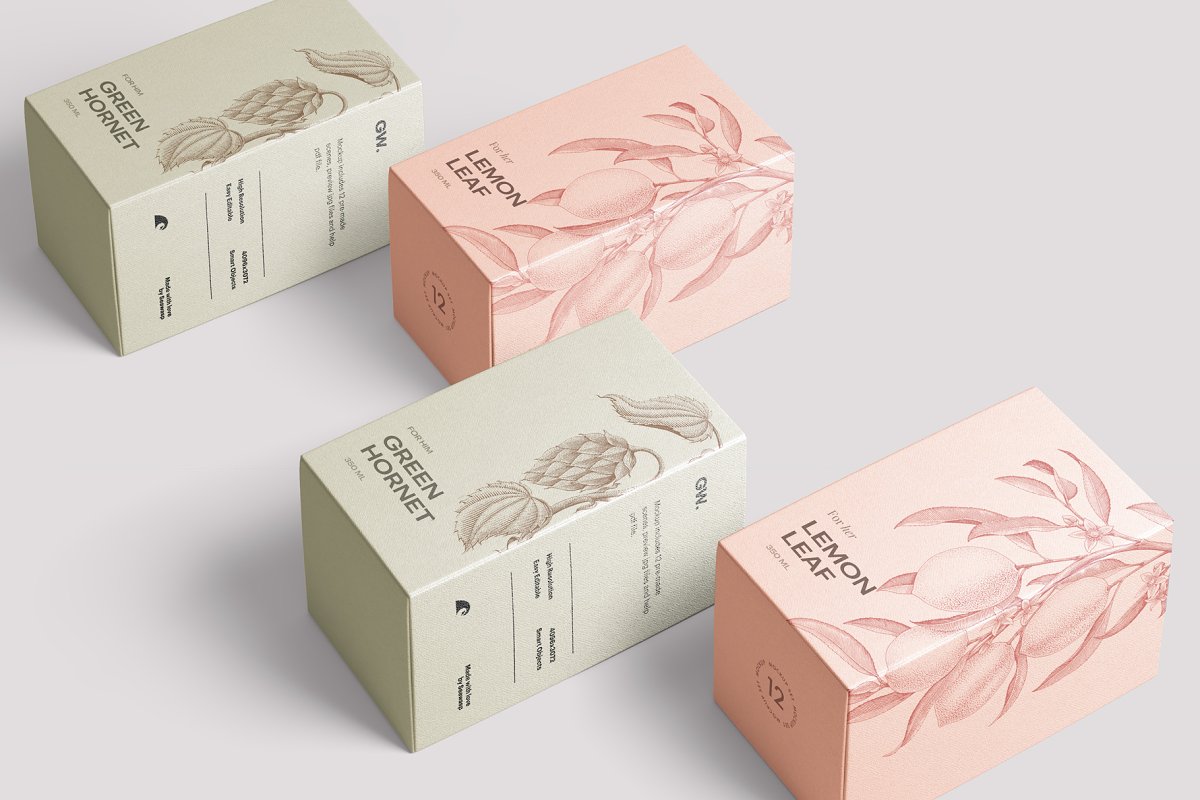This photograph features a well-staged arrangement of four tea boxes set against an off-white background. The boxes are artfully staggered on a diagonal, stretching from the upper left to the lower right corner, creating an engaging visual rhythm. Two of the boxes are a delicate matcha green, showcasing illustrations of beer hops and labeled "Green Hornet" with "For Him" text prominently above. The other two boxes are a pink hue, adorned with lemon tree artwork and marked "Lemon Leaf," with "For Her" inscribed on top. Each box's design includes intricately etched plant motifs, and the Lemon Leaf boxes notably feature a circled number "12" at the bottom. The shadows cast by the boxes add depth to the minimalist white surface beneath, emphasizing the product's branding and aesthetic appeal.